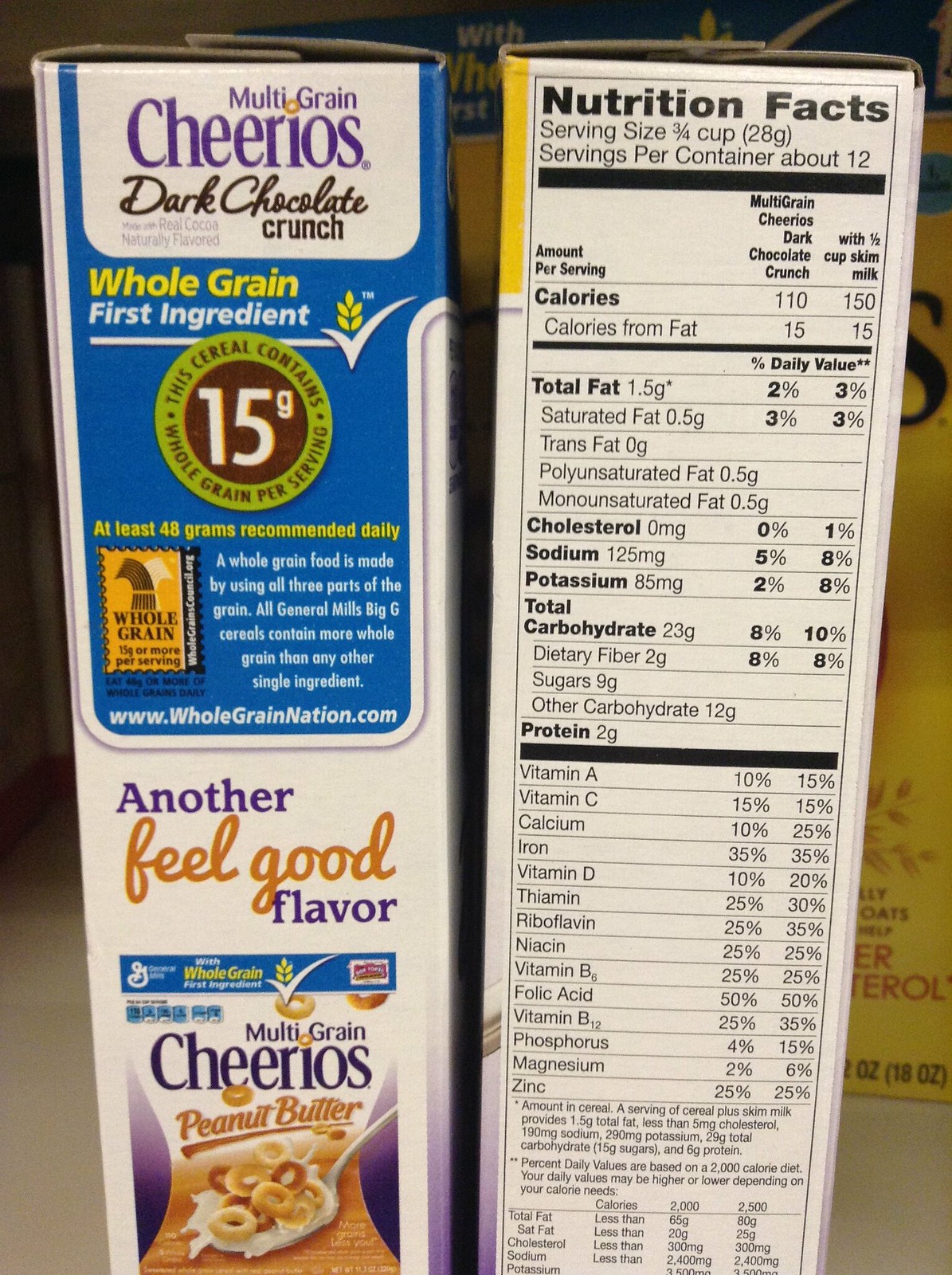This detailed photograph captures the narrow sides of two adjacent cereal boxes. The left box predominantly features a white design with text at the top proclaiming "Multigrain Cheerios Dark Chocolate Crunch." A noticeable blue section highlights "Whole Grain First Ingredient" along with "15 grams of whole grain per serving." Directly below this, the phrase "Another Feel Good Flavor" is displayed above an image depicting the front of a different cereal box, labeled "Multigrain Cheerios Peanut Butter." The right box is dedicated to nutritional facts, presented against an entirely white background with black lettering. It details serving size (3/4 cup or 28 grams), the number of servings per container (about 12), and specifies some nutritional values, including a total fat content of 1.5 grams when paired with half a cup of skim milk. Behind these two front-facing boxes, a glimpse of another cereal box in yellow is visible.